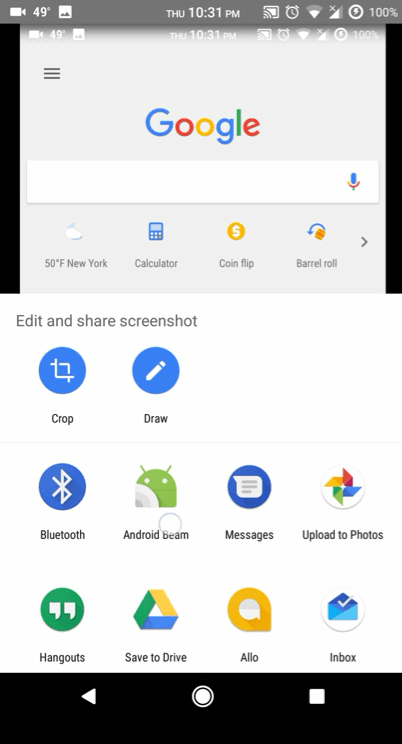A detailed caption for the given image:

"Screenshot captured from an Android device showcasing the Google app interface. The snapshot was taken at 10:31 PM on a Thursday, indicated by the timestamp at the upper section of the screen. At the moment of capture, the device was fully charged at 100% and connected to a charger. The user was utilizing a WiFi connection, as shown by the status bar icons. The notification bar displays a video call in progress, evidenced by the video camera icon in the top left corner, suggesting the user is on FaceTime with someone.

After capturing the screenshot, the Android device presents multiple actions for processing the image. The options visible include editing the screenshot through in-app icons for cropping and drawing, sharing via Bluetooth, sending through the Messages app, uploading to Google Photos, sharing via the Hangouts icon, saving to Google Drive, utilizing the Allo app, and sending via the Inbox app.

Additionally, the screenshot shows that the user has recently swiped a notification away prior to taking the screenshot, emphasizing the captured moment's focus on the available post-screenshot functionality."